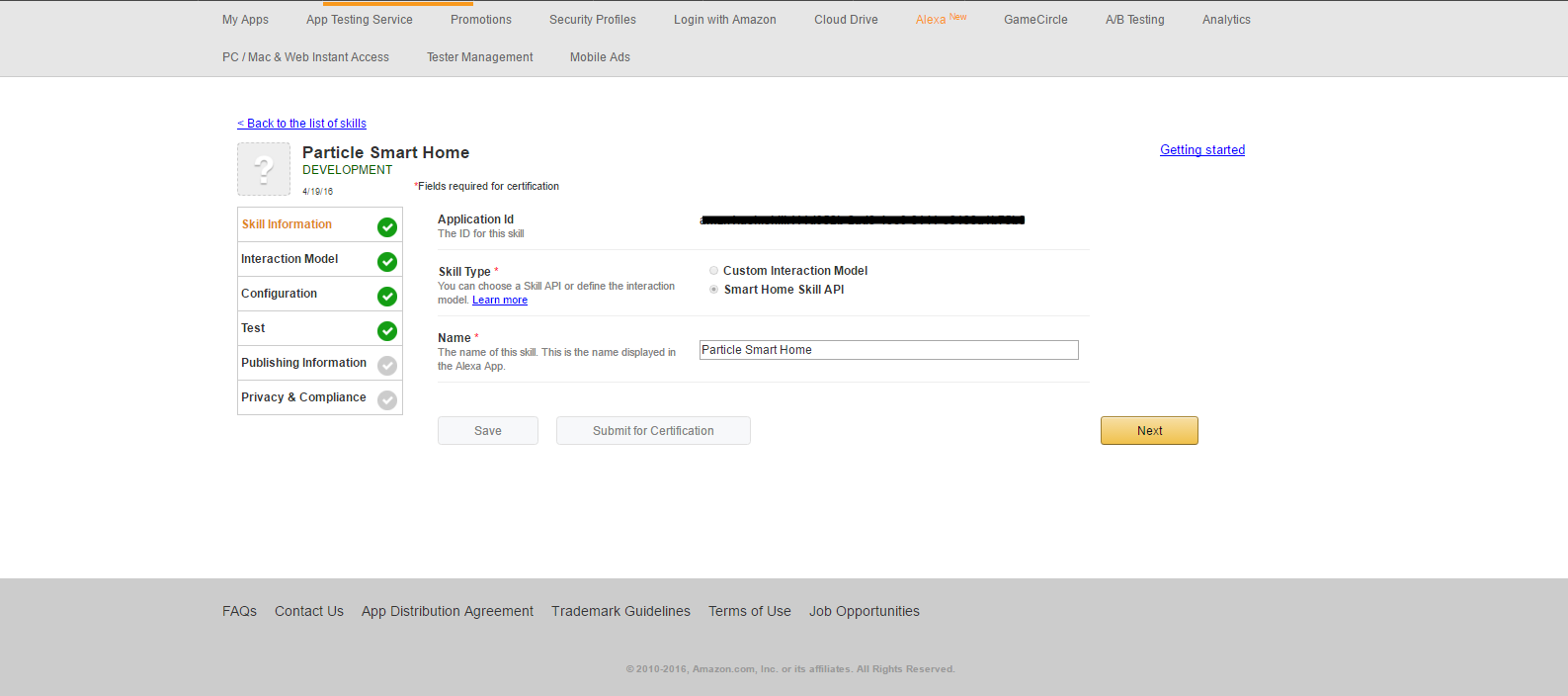This is an image of a website featuring a light gray header and footer. The header contains small, blurred words arranged in two rows. From the top left, the visible words include "My Apps," "Services," "Protection," and "Login," with some text written in orange.

The middle section of the website has a white background with underlined blue text on the left. Adjacent to this is a gray box with a white question mark inside. To the right, there is a title that reads "Particle Smart Home Development," with "Particle Smart Home" in black and "Development" in green. Below this title, orange and black text is accompanied by green circles with white check marks next to certain words.

Further to the right, additional small black text and a search bar are visible. In the top right corner of this white section, "Getting Started" is written in blue. At the bottom right, there's an orange button labeled "Next" in black letters.

The gray footer contains more text, including "FAQs," "Contact Us," "App Distribution Agreement," "Trade something," "Terms of Use," and "J35 Operation Opportunities."